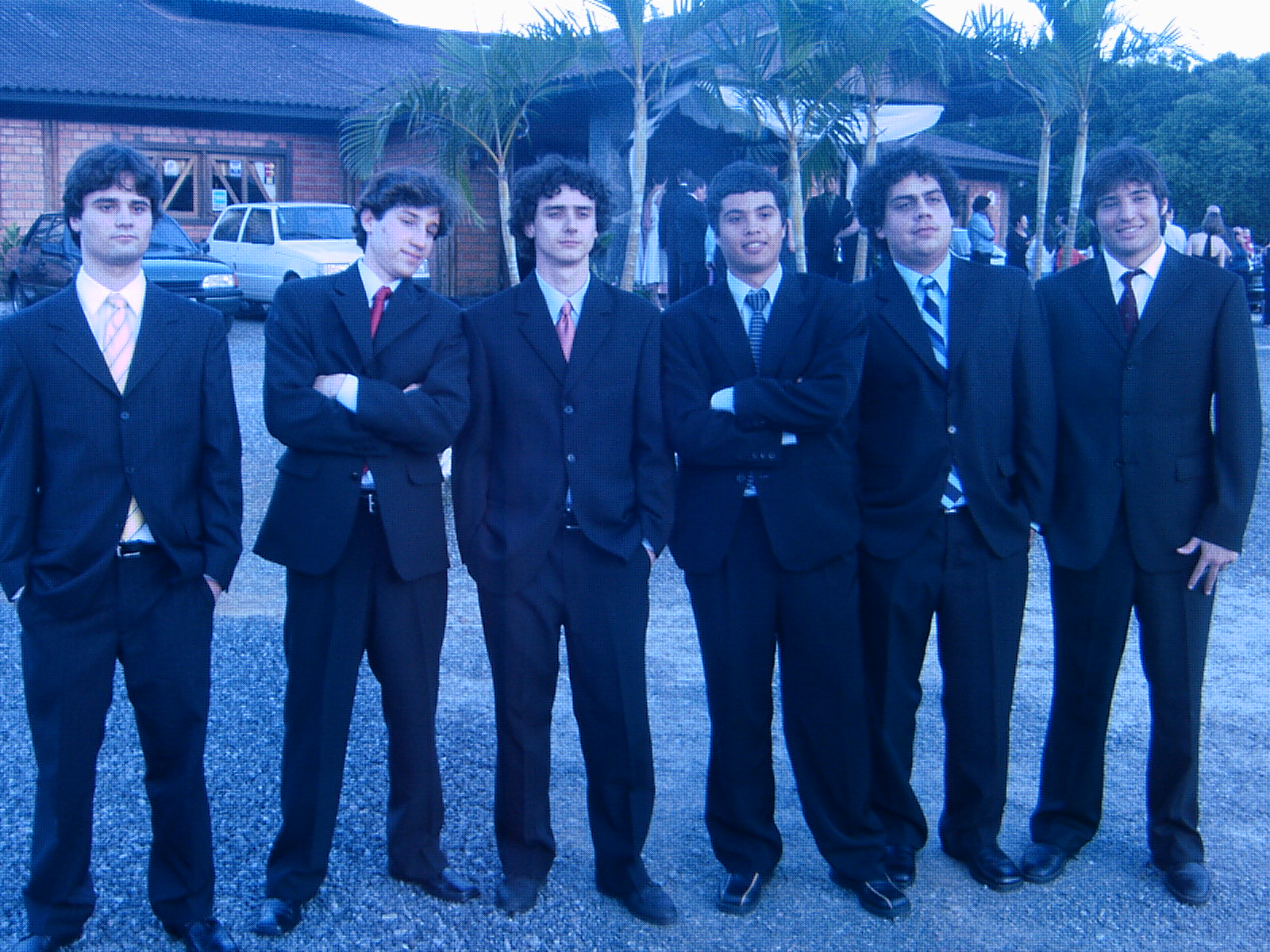The image captures six young men standing in a line, dressed in black suits with black dress shoes and various colored ties. They appear to be late teenagers or in their early 20s, each exuding a sense of formality. Their ties present a splash of color: an orange tie with blue stripes, a red tie, a blue tie, a blue tie with black stripes, and a black tie. The young men have dark hair and are smiling, contributing to a cheerful atmosphere.

They are positioned outside a large brick building with a black roof and an overhanging awning, possibly a venue for a formal gathering such as a wedding reception or prom. Palm trees can be seen near the entrance, giving the venue a tropical, almost Hawaiian feel. The photograph has a slight blue tint, suggesting it might be an older or slightly washed-out image. Several cars and formally dressed individuals are visible in the background, further indicating the setting of a celebratory event.